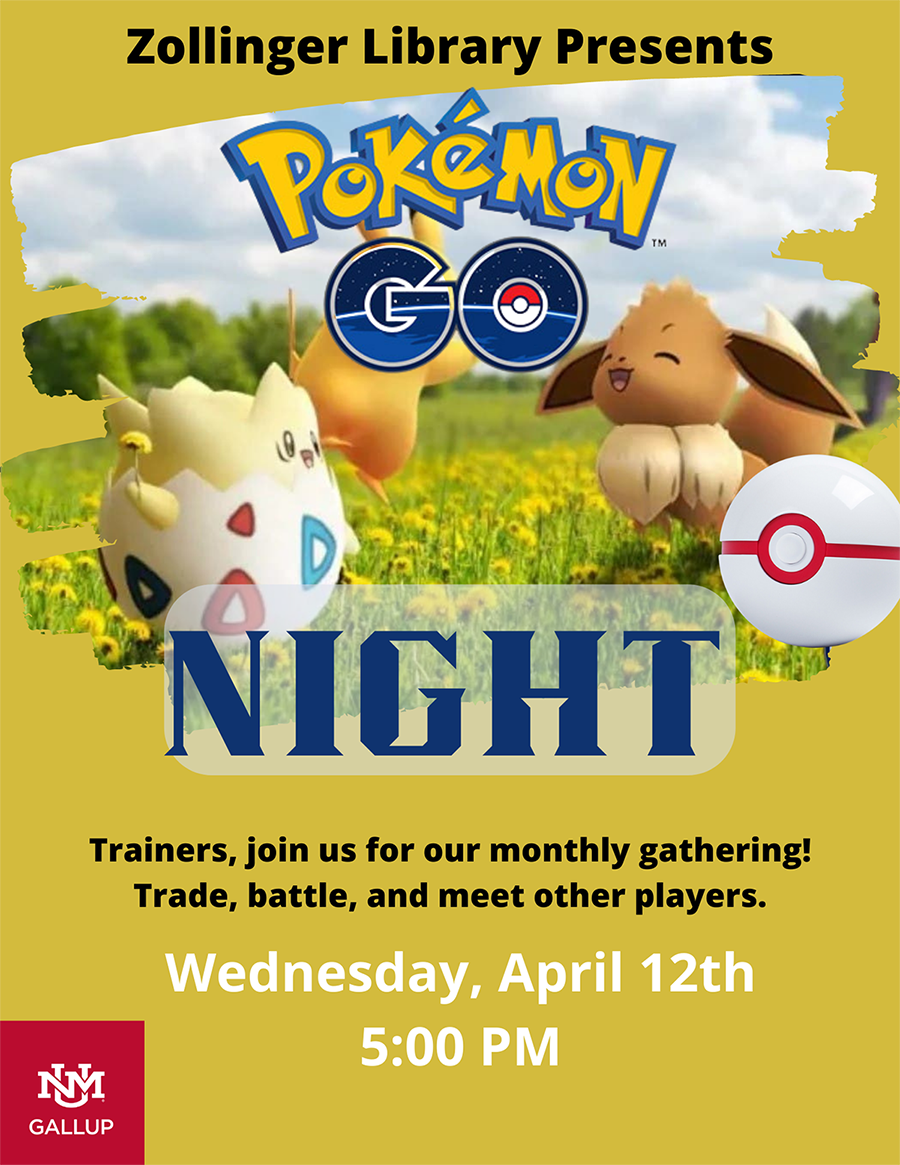The flyer features a dark yellow background with text and images promoting an event at the Zollinger Library. At the top, "Zollinger Library Presents" is written in bold black letters. Below this header, there are images of three Pokémon. On the left is Togepi, depicted in its characteristic eggshell with red and blue triangular patterns. To its right is a Pokémon resembling a brown puppy with long hanging ears and white hair around its chest, which appears to be Rockruff.

To the right of these two, partially obscured by the text, is a yellow Pokémon that seems to be Pikachu. The words "Pokémon Go" cover a large part of its face, but its distinct yellow body is still visible.

Underneath these images, there is a partially transparent white rectangle with "NIGHT" written in bold blue capital letters. Below that, the text in black reads: "Trainers, join us for our monthly gathering. Trade, battle, and meet other players."

Further details state the event will occur on Wednesday, April 12th at 5 p.m.

In the bottom-left corner, there is a red square with a logo in white featuring the overlapping letters "N," "M," and a "U." Below the logo, the word "Gallup" is written in white letters.